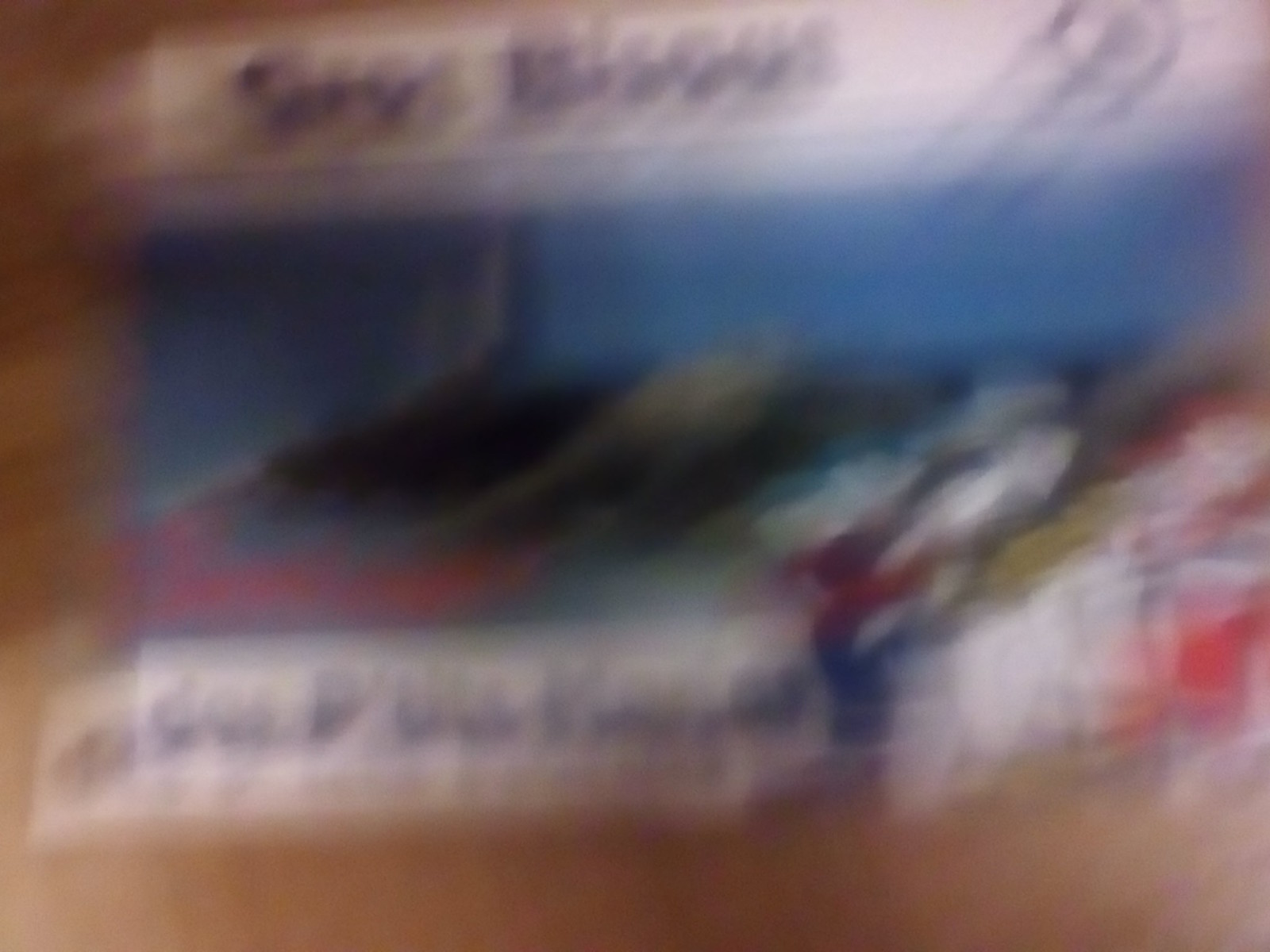The image is extremely blurred and appears to be taken indoors, showcasing several items laid out on a counter. In the foreground, there is a long, rectangular white box with dark-colored writing on the side. This box features a tab, suggesting it is designed to hang on a rack. Behind this box, a larger rectangular object with a white top and dark writing is visible, though its exact nature is indiscernible. Below the white part, there is a blue rectangular section that seems to be the bottom of the box with the white lid. Additionally, several other objects, possibly including an adjustable wrench and spark plugs, are diagonally arranged and situated in the right-center part of the image. However, due to the blurriness, the specific details and types of these items are difficult to determine.